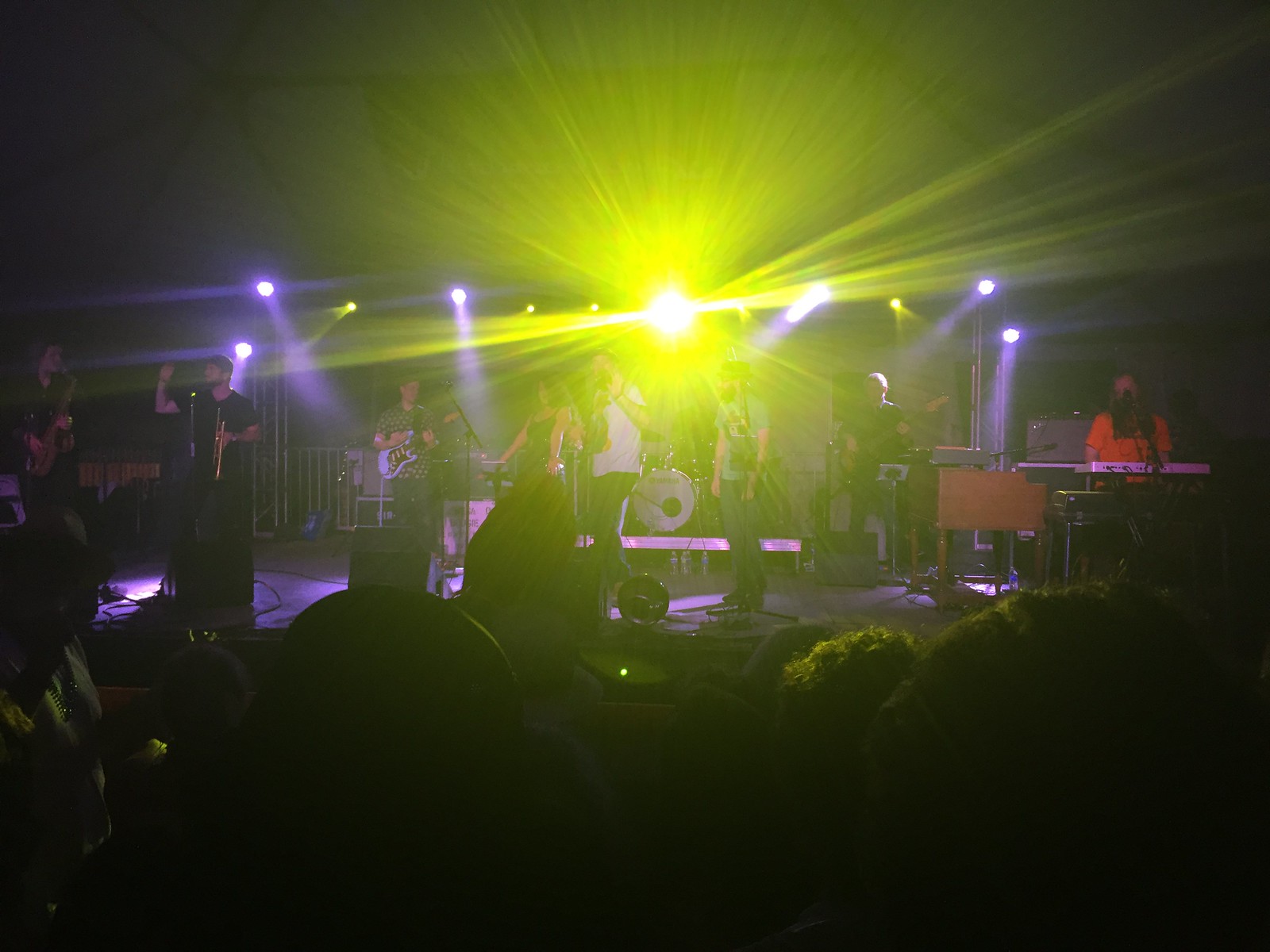The image is a dimly lit, horizontally aligned rectangular photograph of a concert. It features a stage packed with at least seven to eight band members mid-performance, enveloped in a mix of purple lighting and a strikingly bright yellow spotlight in the center that bursts outward with sun-like rays. Below this intense spotlight, the band is arranged across the stage. 

On the far right, a female musician in an orange t-shirt is playing a keyboard or synthesizer. Next to her, a guitarist dressed in a black shirt is seated. Three singers are positioned at the front; one is a woman in a black dress or tank top, flanked by two men. To the left of them, another guitarist, notably in a blue shirt with polka dots, holds his instrument.

Further to the left, a man in a green shirt stands near a microphone, appearing to engage with the audience. Another musician in a white t-shirt seems to be waving, while a man in a black shirt, perhaps playing a horn or trombone, also acknowledges the crowd. Finally, a saxophonist is present on the far left. The bottom of the image shows the dark silhouettes of the audience’s heads, indicating the photo was taken from within the crowd.